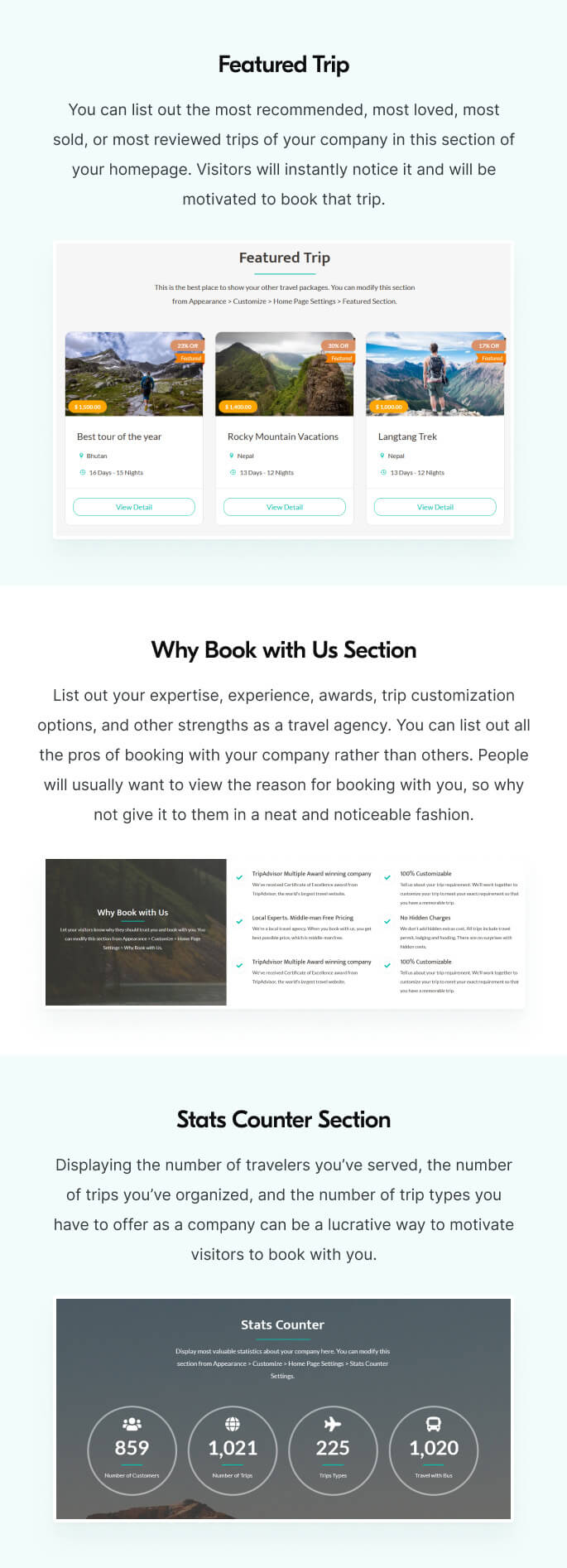This image represents the layout of a travel agency's homepage, meticulously designed to entice potential customers. 

**Header Section:**
- At the very top, bold black text prominently displays "Featured Trip".
- Below the header, a small paragraph in dark gray font explains the purpose of this section: "List out the most recommended, most loved, most sold, or most reviewed trips of your company here. Visitors will instantly notice it and be motivated to book that trip."

**Featured Trip Options:**
- A highlighted box with the label "Featured Trip" stands out, containing three photographic options.
- Each of the three images features stunning mountain landscapes; two of them include a person centrally positioned, emphasizing the adventure and personal experience offered by these trips.

**Why Book with Us Section:**
- Following this, bold black text introduces the "Why Book with Us" section.
- An accompanying paragraph elaborates: "List out your expertise, experience, awards, trip customization options, and other strengths as a travel agency. Showcase all the pros of booking with your company rather than others. Providing this information in a neat and noticeable fashion can significantly influence potential clients."

**Informative Blocks:**
- Below this text are three concise blocks of information, each highlighting a unique selling point of the travel agency.

**Stats Counter Section:**
- Another prominent black text header introduces the "Stats Counter" section.
- A subsequent paragraph highlights the importance: "Displaying the number of travelers you've served, the trips you've organized, and the variety of trip types you offer can be a compelling way to encourage bookings."
- This section includes a stat counter with the following figures:
  - 859 travelers served
  - 1021 trips organized
  - 225 trip types available
  - 1020 (possibly denoting another category such as positive reviews or repeat customers)

This structured layout effectively communicates the agency's offerings, benefits, and credibility, designed to capture and retain the interest of site visitors.